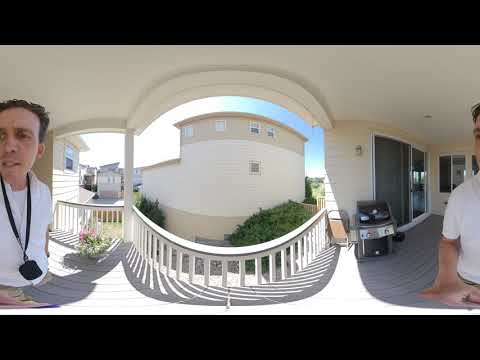In a panoramic fisheye image of a patio, a man with short brown hair stands prominently on the left side, partially reappearing on the right side. He wears a white shirt and a black lanyard with a rectangular object hanging from it. The image captures his concerned expression, with his eyes staring off and his mouth slightly open. The patio area features a white railing, suggesting an upper floor with a view overlooking a courtyard with shrubbery. On the right side, there is a closed barbecue grill, sliding glass doors, and a window, half of which is dark and the other half open. A folded chair leans against the wall nearby. Bright sunlight casts clear shadows of the railing, emphasizing the sunny day. Adjacent to the man, a vase of pink flowers adds a touch of color to the scene.